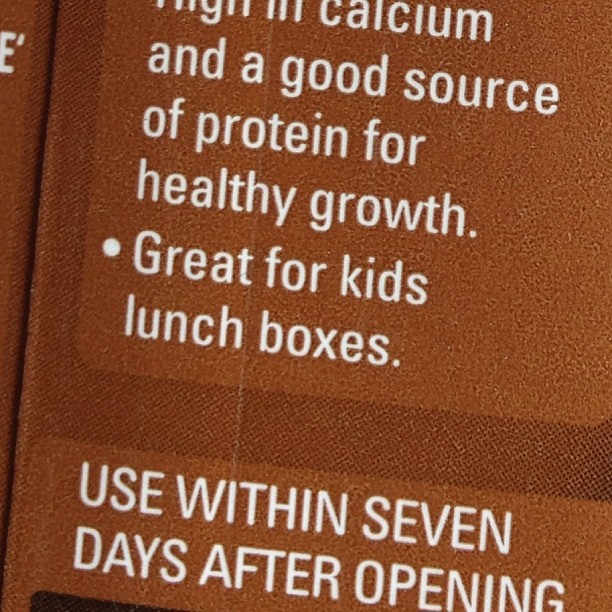A close-up photograph capturing a portion of a food product package against a black, textured background, likely cardboard. Prominently displayed in white and brown lettering, the packaging advises consumers to use the product within seven days after opening. At the top of the image, text highlights the product's nutritional benefits, emphasizing that it is high in calcium and a good source of protein, contributing to healthy growth. It also mentions that the product is ideal for children's lunchboxes. Some partially visible text on the left side of the frame hints at additional information, though it is too obscured to read clearly. The overall texture and format suggest that this is a boxed item specifically designed for convenience in lunch preparation.